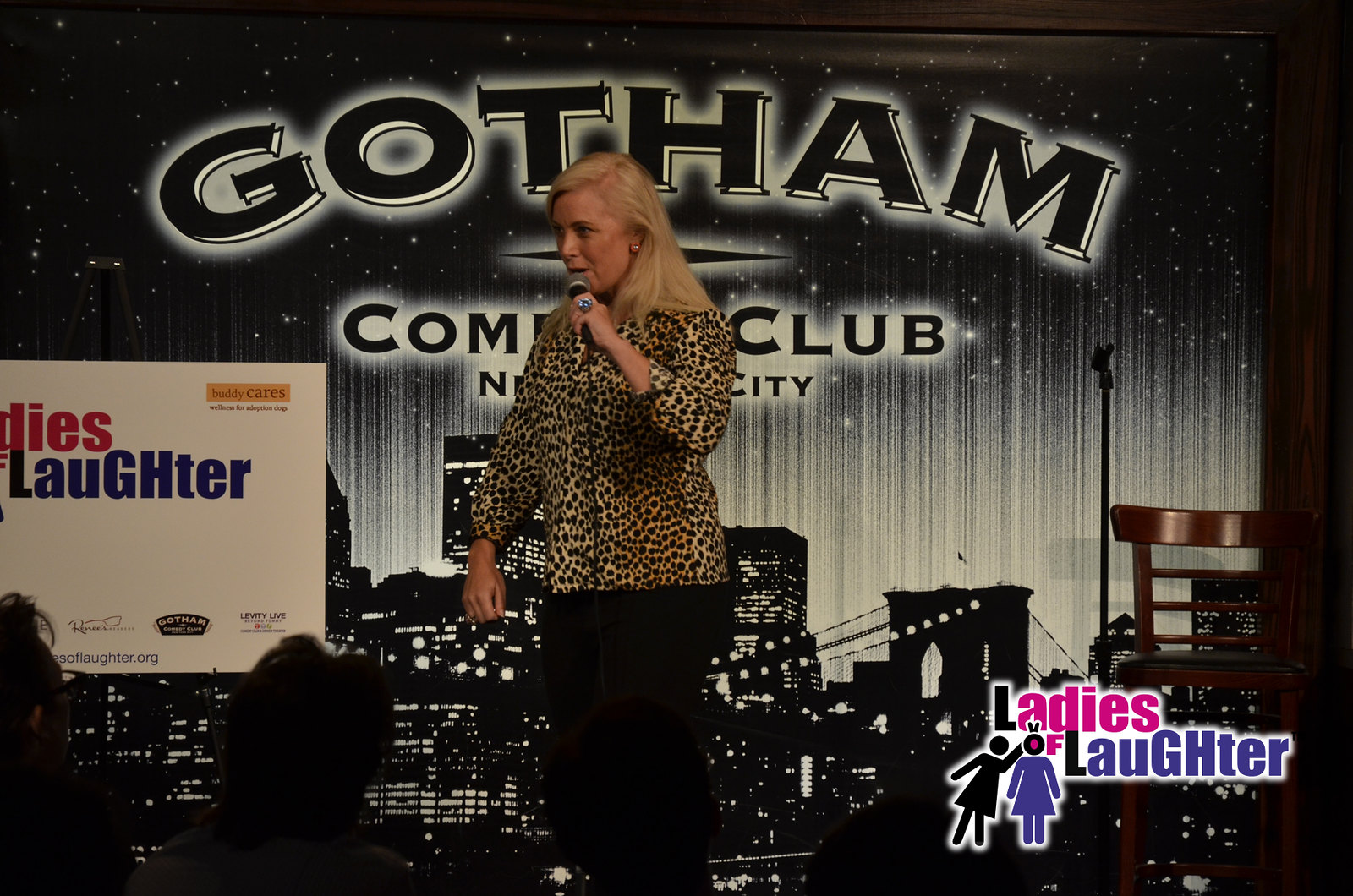The image captures a stand-up comedian performing at the Gotham Comedy Club in New York City. The background features a black-and-white cityscape with the bold, white-shadowed letters of "Gotham" prominently displayed at the top, followed by "Comedy Club" below, partially obscured by the comedian. In the lower right corner, there's a watermark logo for the "Ladies of Laughter Comedy" event, featuring the words "Ladies" in pink and "Laughter" in purple with accompanying stick figures. The left side of the stage shows a partially visible white poster adorned with pink and purple text, likely promoting the event or its sponsors. 

The comedian, a blonde woman who appears to be in her late 40s to late 50s, stands at center stage, engaging with the audience. She is dressed in a long-sleeved cheetah-print shirt and black pants, holding a microphone in her left hand, adorned with a noticeable ring. To her right, there is a wooden chair and a mic stand. Audience member silhouettes are visible at the bottom of the image, hinting at the crowd's presence and engagement.